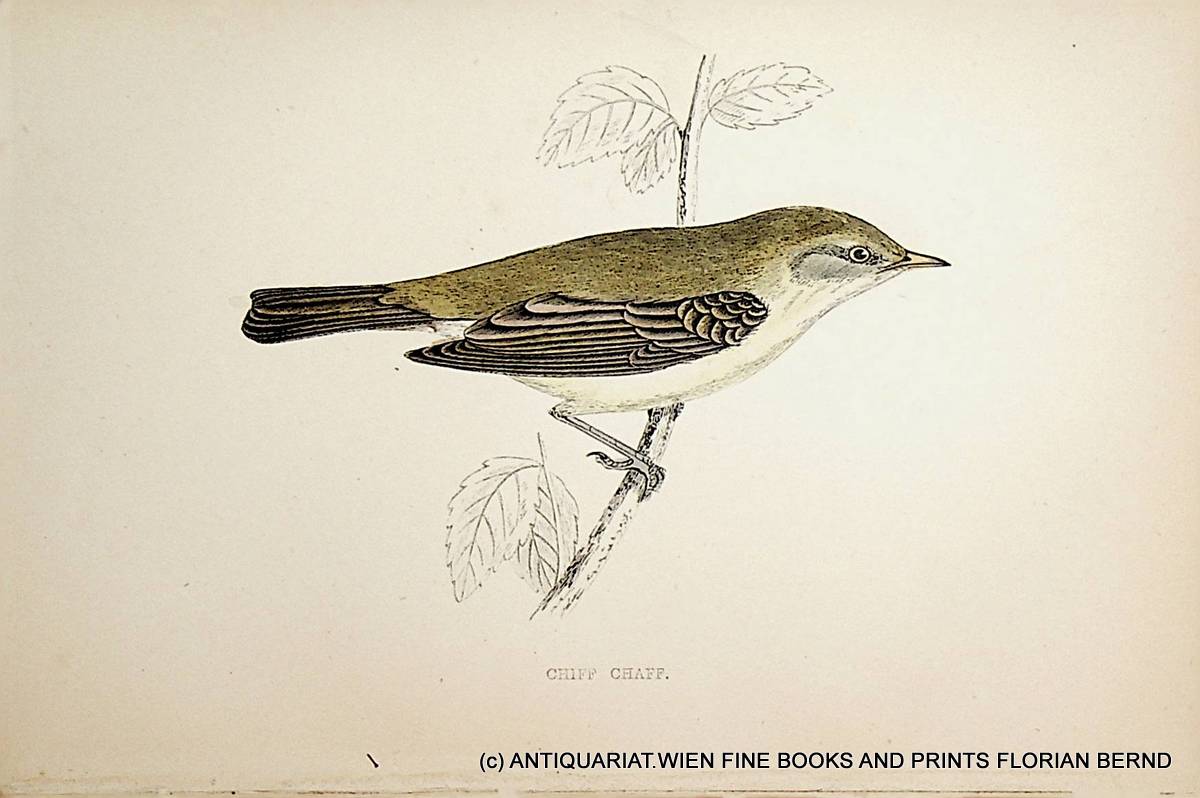This is an illustration from a book featuring a bird perched on a branch. The bird, identified as a "Chiff-Chaff," is rendered in browns and greenish yellows, with its feathers detailed in darker and lighter shades. The chest is lighter, almost white or off-white, while the back and face exhibit a greenish-yellow hue. The tail and wings are darker, contributing to the bird's textured appearance. A subtle stripe runs from the bird's beak, past its eye, and toward its back, adding to the intricate details.

The background of the illustration is an old-looking, beige, antique-style paper. The branch the bird stands on is sketched in black and white, accompanied by a few detailed leaves. One of the bird's legs is wrapped around the branch, enhancing the lifelike quality of the drawing.

At the bottom of the image, the text "C ∙ Antiquariat:wein Fine Books and Prince Florian Bernd" is inscribed, along with the bird's name "Chiff-Chaff" in a typewriter-like font. This text suggests a potential source or credit for the illustration and hints at the antiquarian nature of the book.